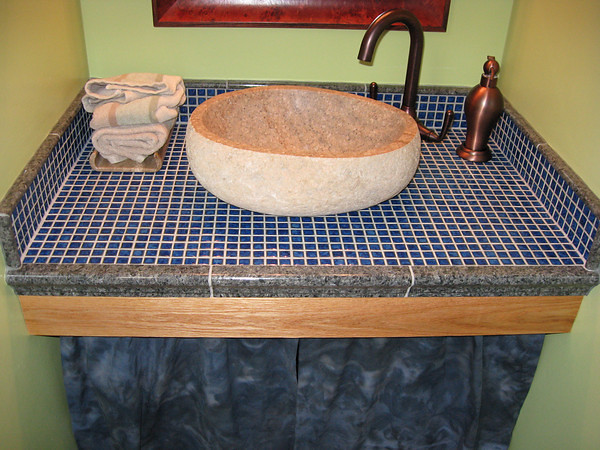This image features a carefully designed bathroom vanity with a single sink. The faucet is a polished bronze, exuding a rich, dark brown hue. The countertop surrounding the sink is composed of small, square tiles, adding a textural element to the space. To conceal the plumbing beneath the sink, a black curtain is neatly draped. The bathroom walls are painted a striking lime green, creating a vibrant backdrop. The sink itself is a distinguished stone bowl, with a tan or khaki exterior and a darker tan interior. Positioned to the left of the bowl is a holder stocked with hand towels. On the right side of the bowl, adjacent to the faucet, sits a dark brown soap dispenser that complements the faucet's color, lending a cohesive look to the vanity.